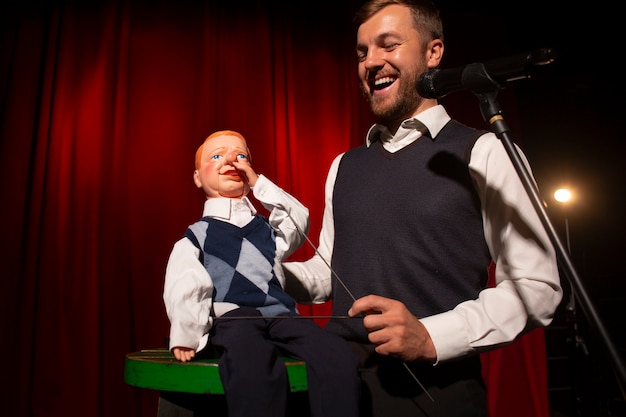In this captivating photograph, a ventriloquist and his puppet are performing on stage in front of a rich red curtain, illuminated by a single spotlight from the right. The ventriloquist, with brown hair, a mustache, and a beard, exudes a joyful energy as he smiles broadly into a microphone. He is dressed in a long sleeve white button-up shirt, black pants, and a plain black vest. 

Standing to his left on a small green stool is his puppet, which bears a striking resemblance to the ventriloquist but features vibrant red hair and blue eyes, along with distinctive rosy cheeks and nose. The puppet is adorned in a white dress shirt, blue slacks, and an eye-catching blue argyle sweater vest. The ventriloquist's right hand expertly controls the puppet, positioning its left hand up towards its mouth, enhancing the lifelike interaction between them. 

The scene is set against a classic stage backdrop, evoking a timeless performance atmosphere.